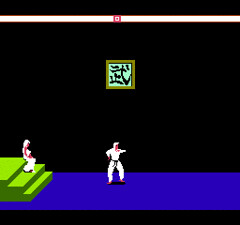This color screenshot, presumably from an older and unknown video game, showcases blocky and pixelated graphics characteristic of early gaming eras. The scene is set in a dark blue environment with a green staircase situated on the right side. A character dressed in white is descending the staircase. Dominating the center of the image is a figure clad in a traditional karate gi with a black belt secured around the waist, indicating a high level of martial arts proficiency. Near the top of the frame, a green sign adorned with black Japanese characters is visible, though the text is not discernible. The image contains no English text or animals.